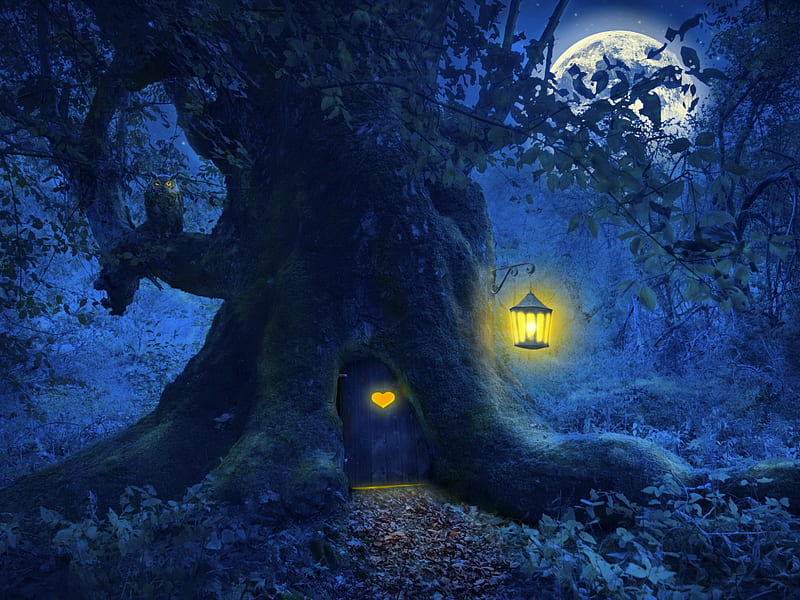The illustration depicts an eerie, nighttime forest scene, perfect for Halloween or a spooky campfire tale. Dominating the image is an old, massive tree trunk, rendered in deep shades of blue and black, with subtle hues of green in the moss. At the base of the trunk, there's an oval-shaped wooden door with a heart-shaped cutout glowing an inviting yellow light, suggesting a tiny creature, like a gnome or fairy, might reside there. On the right side of the trunk hangs a lantern emitting a yellow glow, nestled not too high above the ground. To the left, a thick branch extends out, where a horned owl with piercing yellow eyes perches, casting an imposing presence. In the upper right-hand corner, half-obscured by leaves and branches, a silvery full moon peers through the dark canopy, adding an ethereal glow to the scene. The overall ambiance is deeply atmospheric, shrouded in a mysterious, cold blue tone with warm yellow highlights, enhancing its haunting allure.